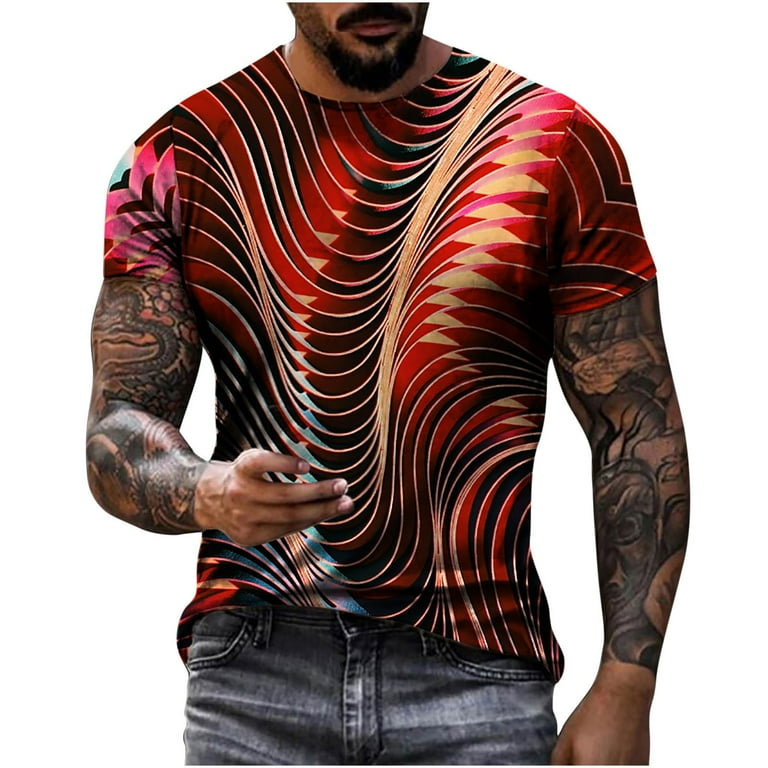This image features a man with a goatee and a full mustache, showcasing his upper body and partial lower body. His skin appears to have an Indian tone. He is adorned with full sleeve tattoos on both arms. The form-fitting shirt he is wearing is particularly striking; it is predominantly red with intricate gold and blue wavy designs that create a 3D effect. The shirt's sleeves add to its unique style, with one sleeve featuring red and black swirls and the other sleeve combining pink, black, and blue swirls. His lower body is clad in gray-blue jeans. The picture is framed, cutting off just below his nose and around his thigh area, enhancing the focus on his detailed tattoos and the shirt’s vibrant patterns. The gold wavy designs on his shirt resemble a chain necklace, adding an extra layer of visual depth to the image.